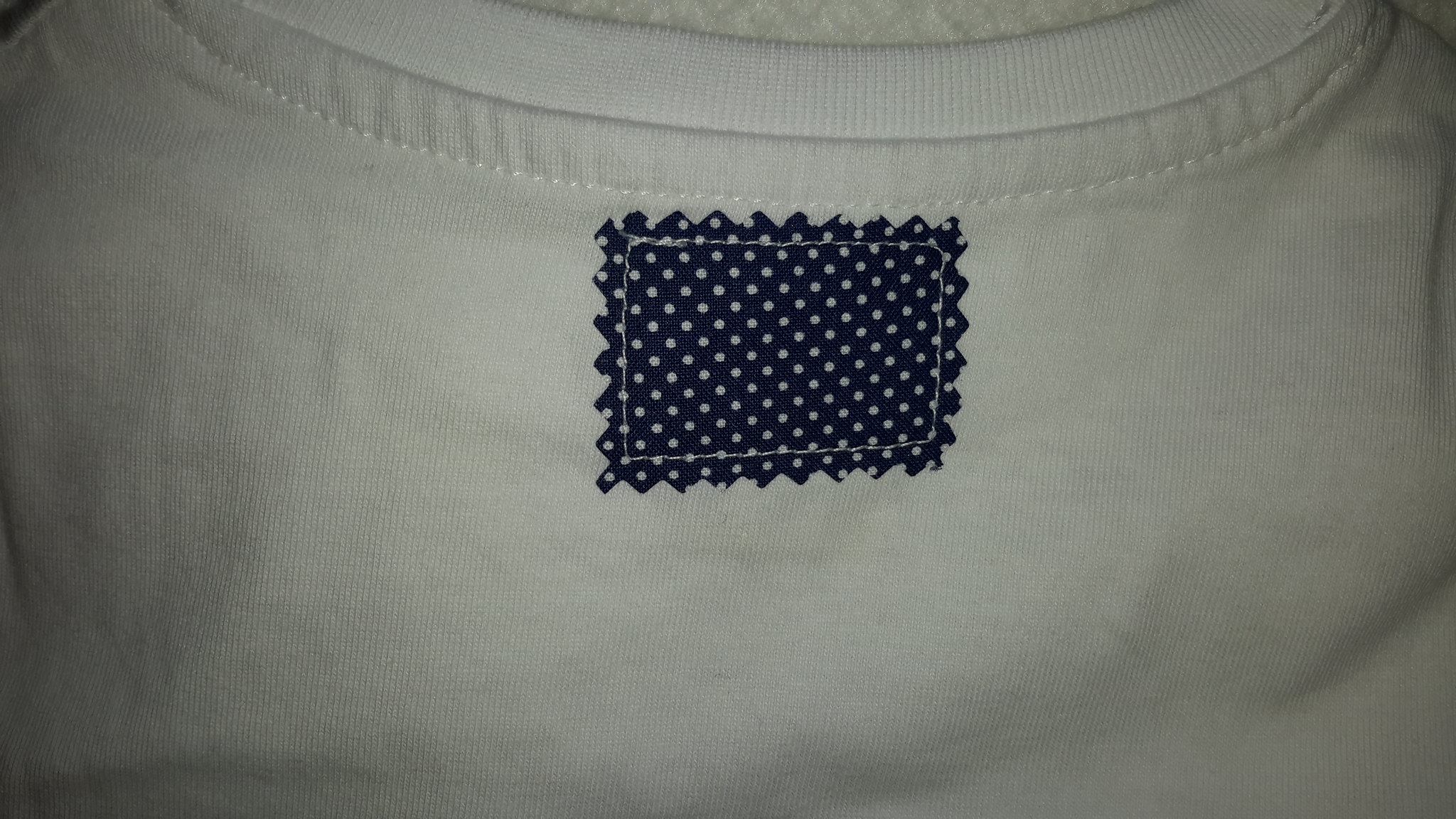The photograph showcases a garment made from white cotton fabric, focusing on its upper portion. The garment appears to be a shirt, specifically emphasizing the rounded neckline which is accentuated with ribbing. The image is a close-up, making it challenging to confirm the entire garment style definitively. Notably, just below the neckline, there is a square area featuring a black background adorned with white polka dots, where a tag would typically be located. This square lacks any text or identifying tag, leaving it unclear whether the tag has been removed or if the design intentionally mimics the appearance of a tag.